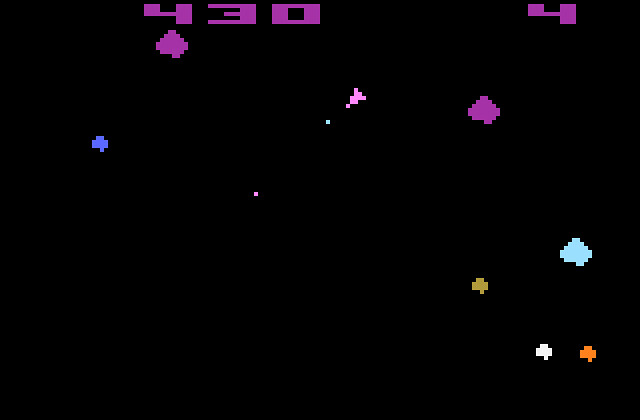The image appears to be a screenshot from a gaming device, featuring a predominantly black background. In the top left corner, the number "430" is displayed in bold purple. Directly below the numeral "4," there is a small purple emblem. Moving slightly further left, there is a tiny blue box with intersecting vertical and horizontal lines inside it. Adjacent to this, a small pink square is visible, and situated above this pink square is a tiny green square.

In the center area of the image, there is a distinct pink diamond-shaped emblem that tapers at both ends and enlarges in the middle. On the far right side of the image, there is a purple diamond-shaped or triangular symbol. Directly above this purple shape, in the top right corner, the numeral "4" is displayed. Beneath this "4," there is a light blue emblem. 

To the left of this blue emblem, a small gold symbol can be seen. In the bottom right corner, there are two small emblems; one white and one orange, positioned side by side.